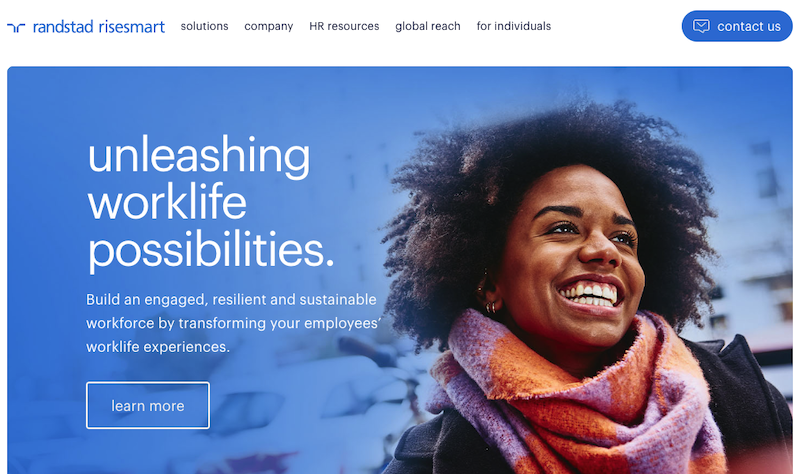In the upper left corner of the image, set against a white background, there's an intricate icon that resembles a series of interconnected lines creating a shape somewhat like a shoulder shrug gesture. Beside this icon, the text reads "Randstad RiseSmart," signifying the name of the company. Below this, there are gray buttons or tabs indicating various offerings of this HR solutions company, specializing in global research and resources for individuals.

On the right, there's a blue circle with white text inside that says "Contact Us," featuring an envelope icon. The background overall shifts to a blue shade, likely a standard design choice.

Dominating the right side of the image, there's a stock photo of a Black person sporting a huge smile and an afro. They are wearing a vibrant blue and orange patterned scarf with a black coat, and they're looking to the right.

On the left side of the image, the white text reads: "Unleashing Workforce Possibilities. Build an engaged, resilient, and sustainable workforce by transforming your employees' workforce experiences." Below this message, there's a white outlined button with the text "Learn More."